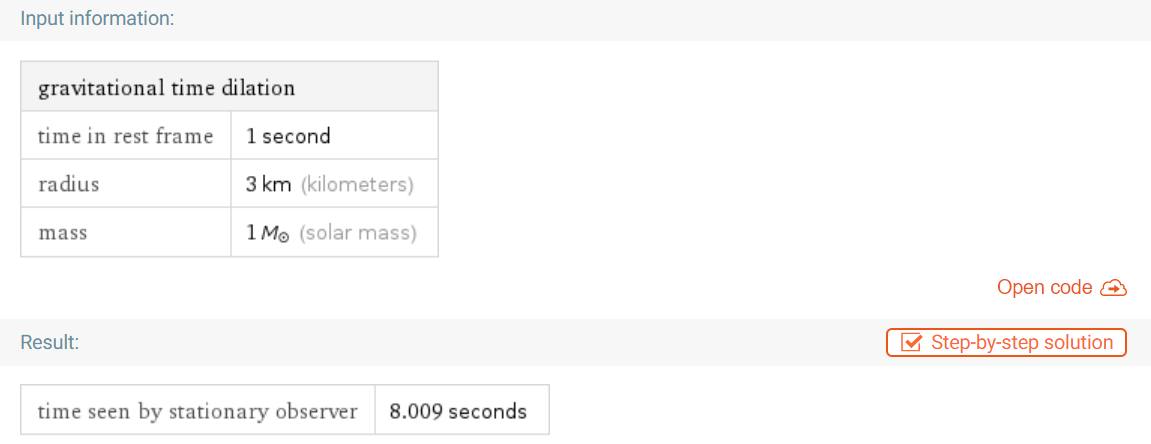The image features a user interface related to gravitational time dilation presented on a light gray bar at the top. In the upper left corner, it displays input information. Below this section, a chart is titled “Gravitational Time Dilation” highlighted on a light gray background. The left column of the chart lists parameters such as “Time in rest frame” followed by “Radius” and “Mass.” Corresponding to these parameters on the right column are “1 second,” “10 km,” and “1 solar mass” respectively. A circle icon next to “Mass” visually represents the concept of a solar mass. 

Beneath this chart, a gray strip showcases results in green text. Adjacent to it, on the right, a button with a white background and a red outline displays the text “Step by Step Solution” in red font. This button features a red checkmark inside a red box preceding the text. Above it, another button featuring an open code icon—a cloud with an arrow pointing right—also in red font, is similarly outlined in red. It seems there could be some irregularity with the outline, suggesting it might have been edited afterward.

Lastly, below these elements, the display details that the “Time seen by stationary observer” is “8.009 seconds” in green text on the gray strip.